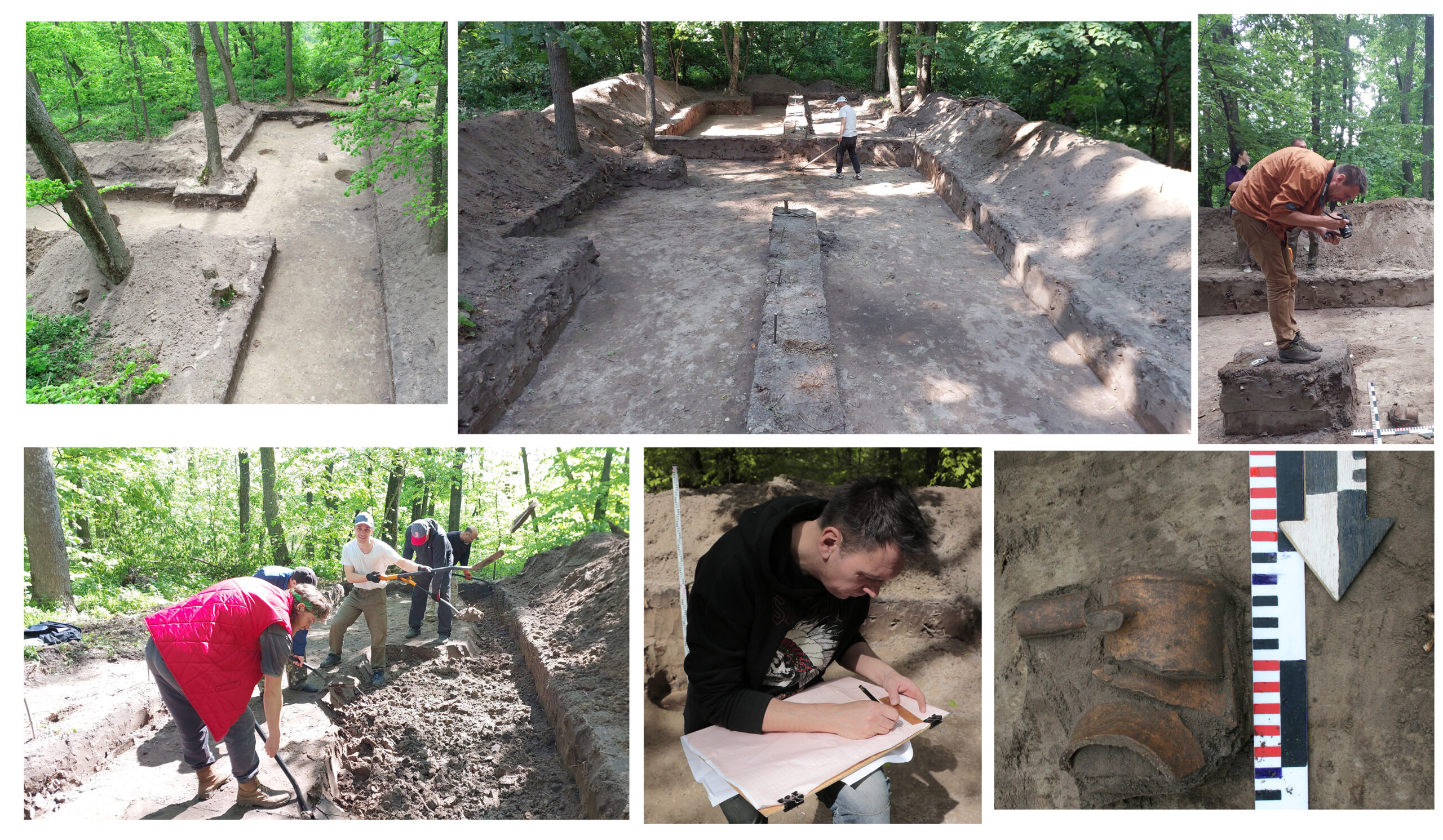A detailed collage capturing an archaeological excavation project unfolds across six distinct photographs. In the upper left image, the initial stages of excavation are evident, as researchers carefully begin their work in a densely wooded area. The second photo provides a deeper perspective into the excavation site, revealing partially exposed walls and two men busily engaged in their tasks, framed by surrounding foliage. The third image on the top row portrays a solitary man standing on a mound within a pit, methodically photographing marker sticks that document specific points of interest.

Transitioning to the lower left corner, three archaeologists are diligently excavating a pit, skillfully using shovels to unearth artifacts near a prominent wall, suggesting this might be a significant structural part of the site. The central bottom photograph focuses on a man dressed in a black hoodie, intently taking notes on paper, highlighting the meticulous documentation process essential to archaeological work. Finally, the bottom right image showcases a fragment of broken pottery or earthenware, situated next to rulers and markers for scale. Set against a backdrop of gray soil, the tan-tinged pottery piece offers a glimpse into the material culture of the past, indicating a significant find within the excavation site.